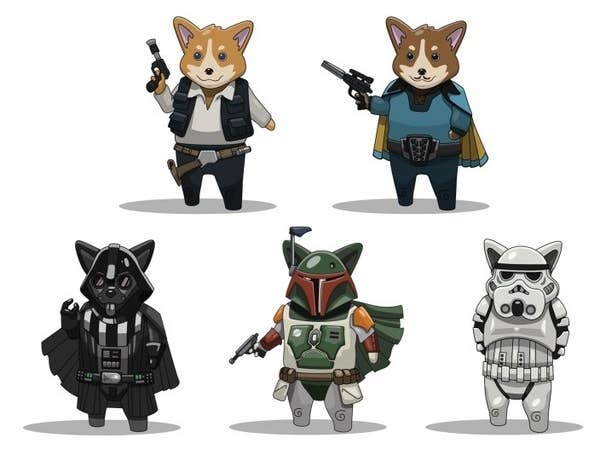This is a charming image of five Star Wars characters reimagined as corgis in a detailed cartoon drawing style, all set against a white background. At the top left is Han Solo, depicted with a light brown corgi face, wearing his classic vest over a polo top, black jeans, and a distinct gun belt hanging over his right hip. He's holding his pistol confidently in his right hand. To his right is Lando Calrissian, illustrated with a darker-toned corgi face, adorned in a blue shirt, white belt, and brown cape edged with bluish green. He has a longer revolver with a scope and sports a prominent mustache. 

The bottom row features three characters: On the far left is Darth Vader, characterized by a black hood, white and black striped chest, and raised right hand, but with corgi ears peeking above the helmet. In the center is Boba Fett, outfitted in grey and green armor with burgundy accents, including his helmet and gauntlets. He has a pistol in his right hand and bear dog ears above his helmet. Finally, on the bottom right is a Stormtrooper, complete with full grey armor, articulated arms, and corgi ears above the helmet, embodying the character's iconic look. Each of these corgi characters stands on a grey surface, adding a delightful and whimsical twist to the Star Wars universe.